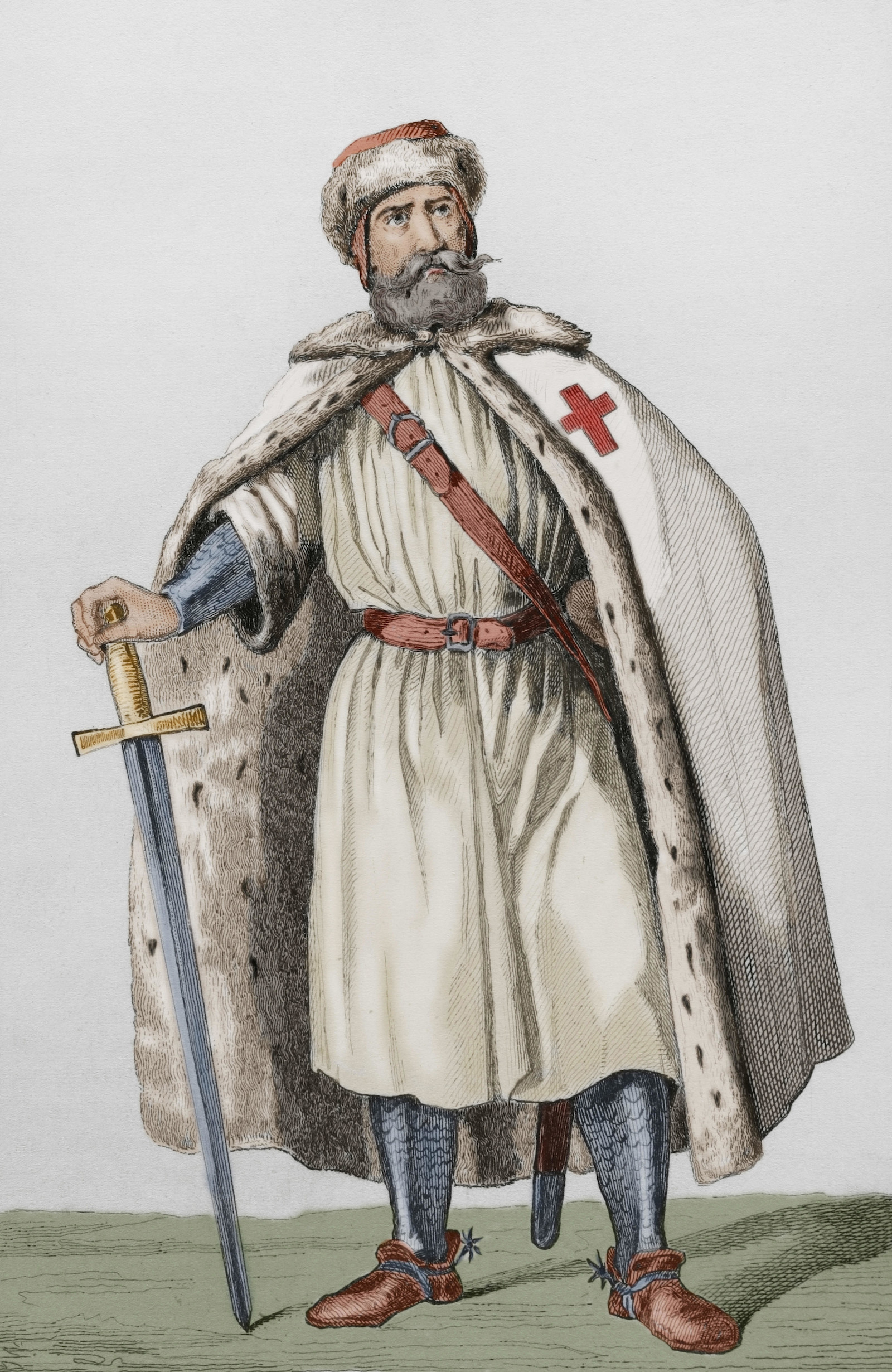This is a meticulously detailed illustration depicting a medieval-era knight, potentially engaged in the Crusades, standing in a solemn, proud pose. The knight, a bearded man with a gray beard and piercing eyes, gazes stoically off to the viewer's right, his left. He wears a white tunic cinched with a brown belt and adorned with a white cloak that features a prominent red cross over his heart. Fur trim lines the cloak's collar and hem, adding to the knightly regalia. His head is crowned with a furred hat, and his hand rests upon the hilt of a sword, which stands tip-down on the ground as if it were a cane. A brown strap crosses his chest, leading to a bag hanging from his hip, its buckle clearly visible. Below the tunic, he is clad in silver chain mail that covers his legs up to just below the knee, where the outline of a scabbard can be seen. He wears brown shoes equipped with spurs, enhancing the period-specific attire. The background is white, contrasting with the green floor, further highlighting the knight's distinguished and heroic stance.